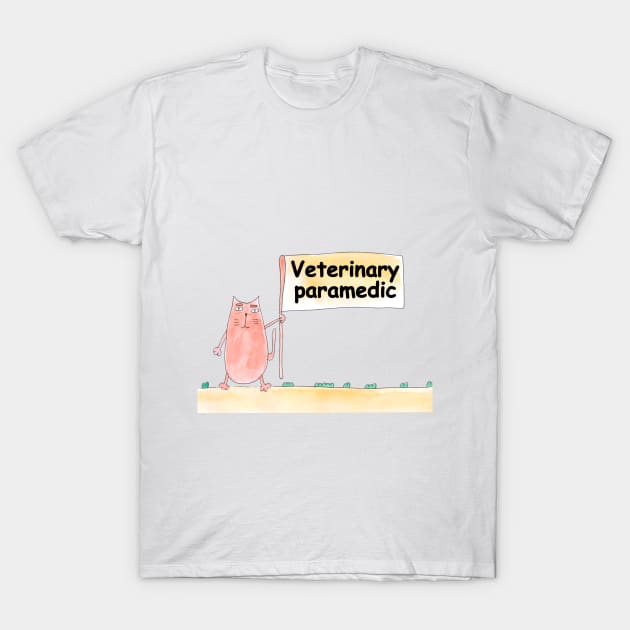This image features a white t-shirt laid flat on a white background, with a whimsical cartoon design at its center. A pinkish-orange cat, illustrated in a simple, penciled-in style, stands on a light yellow rectangular patch suggestive of dirt, adorned with green plants sprouting near its feet. The cat, characterized by its thin legs, an L-shaped tail, and uneven eyes with brownish eyebrows, holds up a yellow flag or sign on a wooden pole. The flag bears the black text "Veterinary Paramedic," with a capital V and lowercase letters for the rest. The cat's face features three short whisker lines on each side, a single line for the mouth, and white eyes with simple black lines for pupils. The t-shirt bears no additional logos, words, or tags.